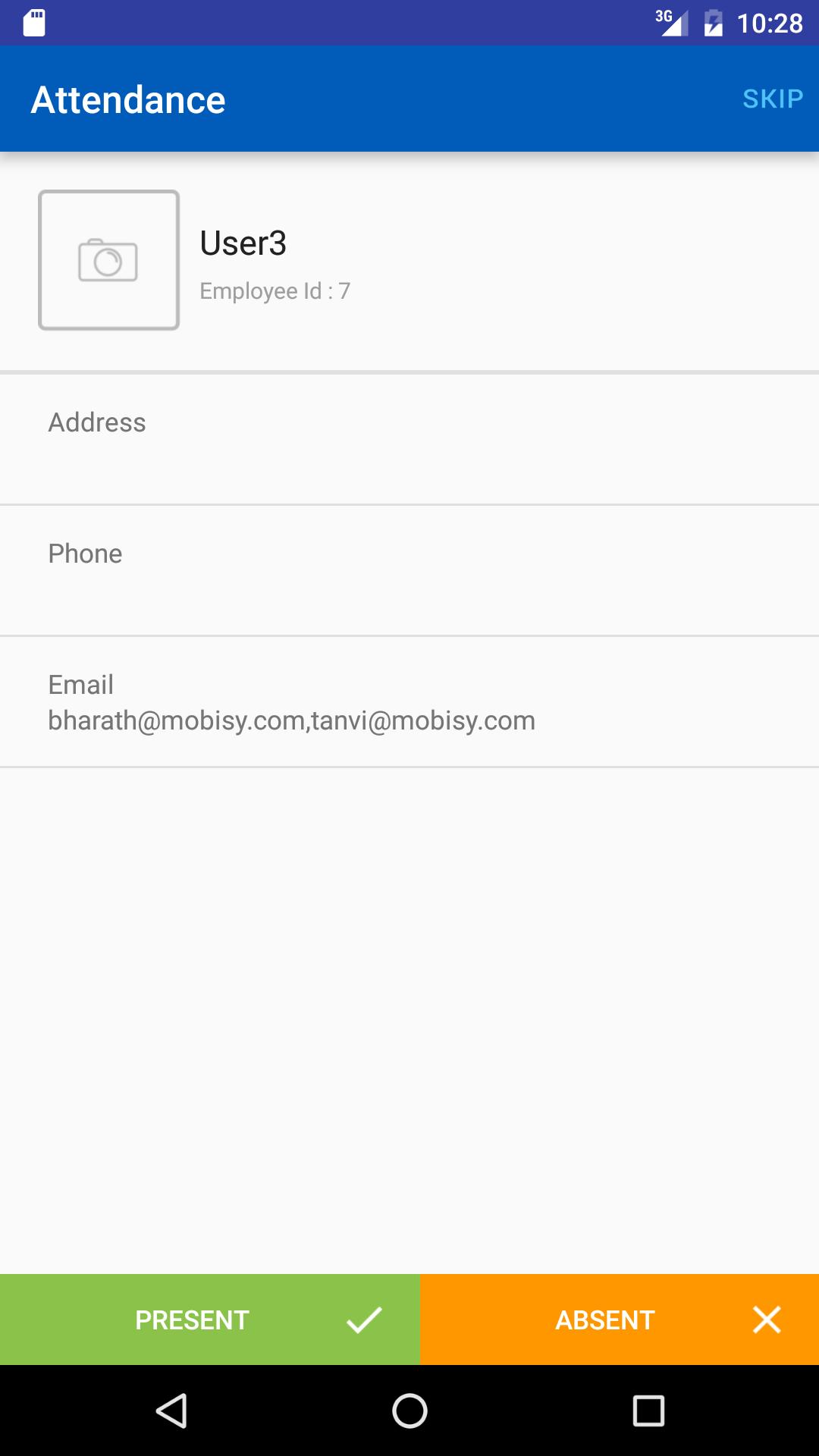A screenshot captured on a phone displays a form interface. In the upper left corner is a file symbol. The upper right corner shows the connectivity service bars, a charging battery icon, and the current time, 10:28. A blue banner at the top bears the word "Attendance" on the left and "Skip" on the right. Below this banner, aligned on the left side, is a square containing a camera symbol. Adjacent to this, on the right side, the text reads "User 3" and "Employee ID 7," separated by a line. Further details include fields labeled "Address," "Phone," and "Email," each with a line for input. The email section includes two addresses: bharath@mobizzy.com, and tanvi@mobizzy.com. Near the bottom of the screen, there are two distinct buttons: a green "Present" button marked with a checkmark, and an orange "Absent" button marked with an X. At the very bottom is a navigation bar on a black background featuring three symbols: a triangle pointing left, a circle, and a square, all with white text indicating their respective functions.